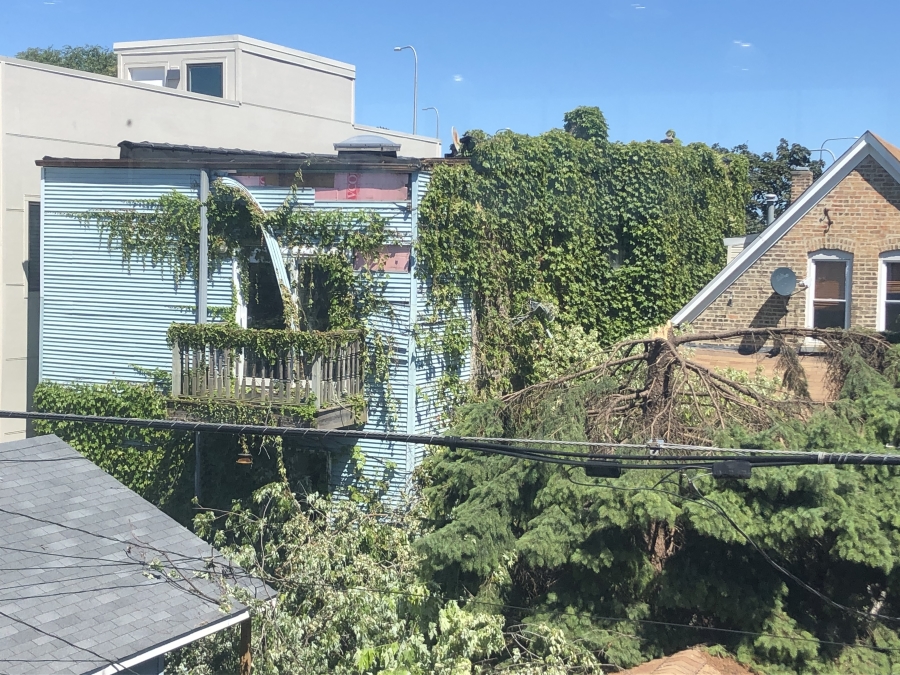This full-color, square photograph captures an outdoor scene on a very sunny day, bathed in natural light. The backdrop features a clear blue sky without any clouds. Dominating the left side of the image is a triangular brick house with two white double-hung windows, a satellite dish, and a pine tree in front of it. The top half of the pine tree appears jagged and broken, likely due to a storm, which has caused the fallen branches to damage an adjacent blue corrugated metal building. The damage is evident as sections of the metal siding are torn away, exposing pink insulation and a damaged wooden deck. Further to the left, partially visible, is an asphalt roof of another house, and in the background, a taller light brown structure rises above the scene. The image also includes electrical and power lines intersecting the view and hints of overgrown vines creeping up the blue building, adding to the complexity of the scene.